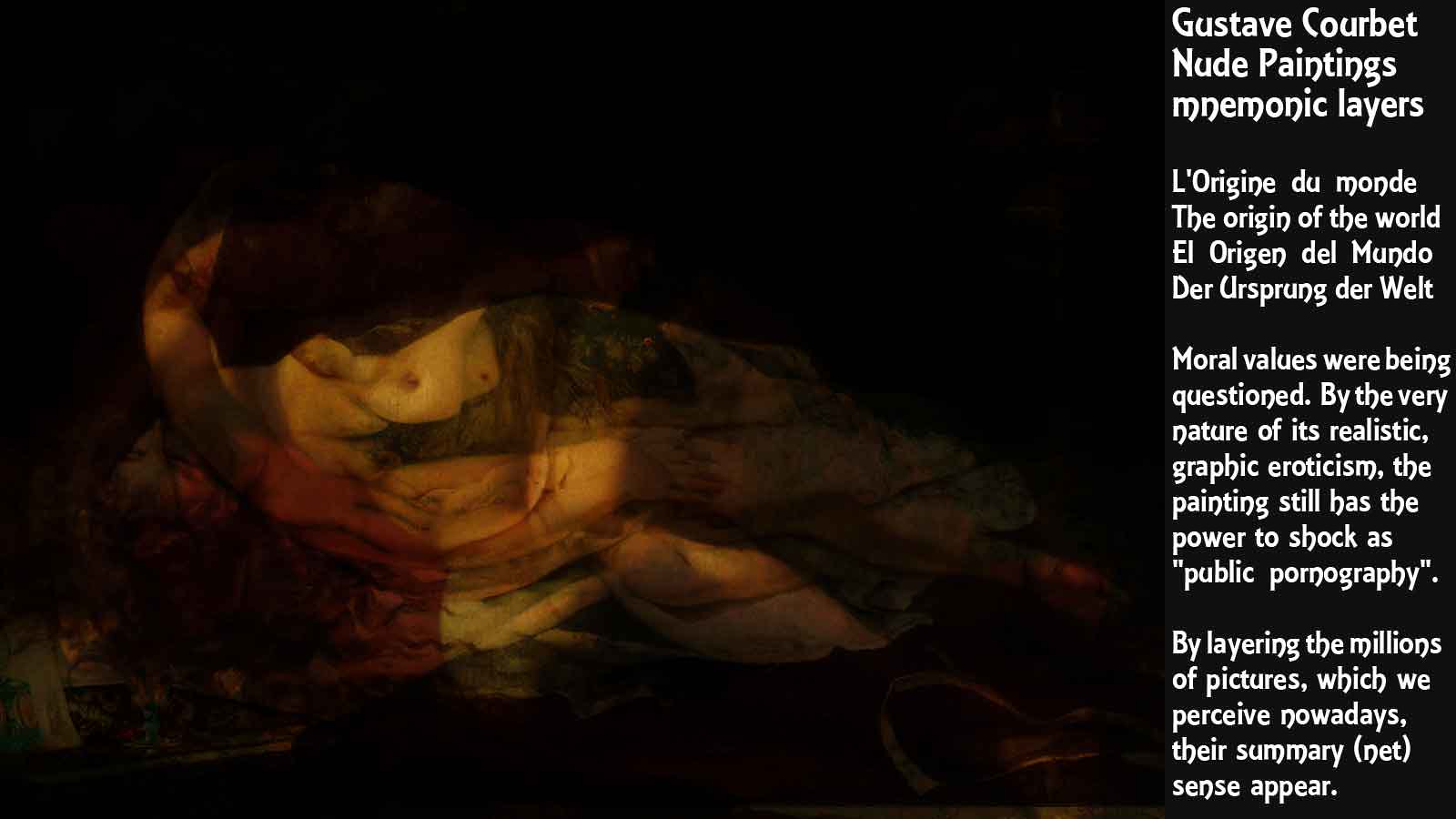The image portrays a striking and complex painting attributed to Gustave Courbet, titled "Mnemonic Layers: The Origin of the World." The painting is predominantly dark, with a stark black background contrasting with flesh-colored, partial depictions of human forms that emerge through layered transparency. Notable elements include visible hands, breasts, knees, and other limbs, suggesting erotic content intertwined in an almost ghostly overlay. The aged and cracked paint evokes an old-world technique, enhancing its antique aesthetic. White text along the right side of the image provides multilingual titles and descriptive commentary, noting, "Gustave Courbet, Nude Paintings, Mnemonic Layers." The text further elaborates, "Moral values were being questioned. By the very nature of its realistic graphic eroticism, the painting still has the power to shock as public pornography. By layering the millions of pictures which we perceive nowadays, their summary net scents appear." This intricate piece evokes a provocative exploration of art, morality, and perception through layers of historical and contemporary imagery.